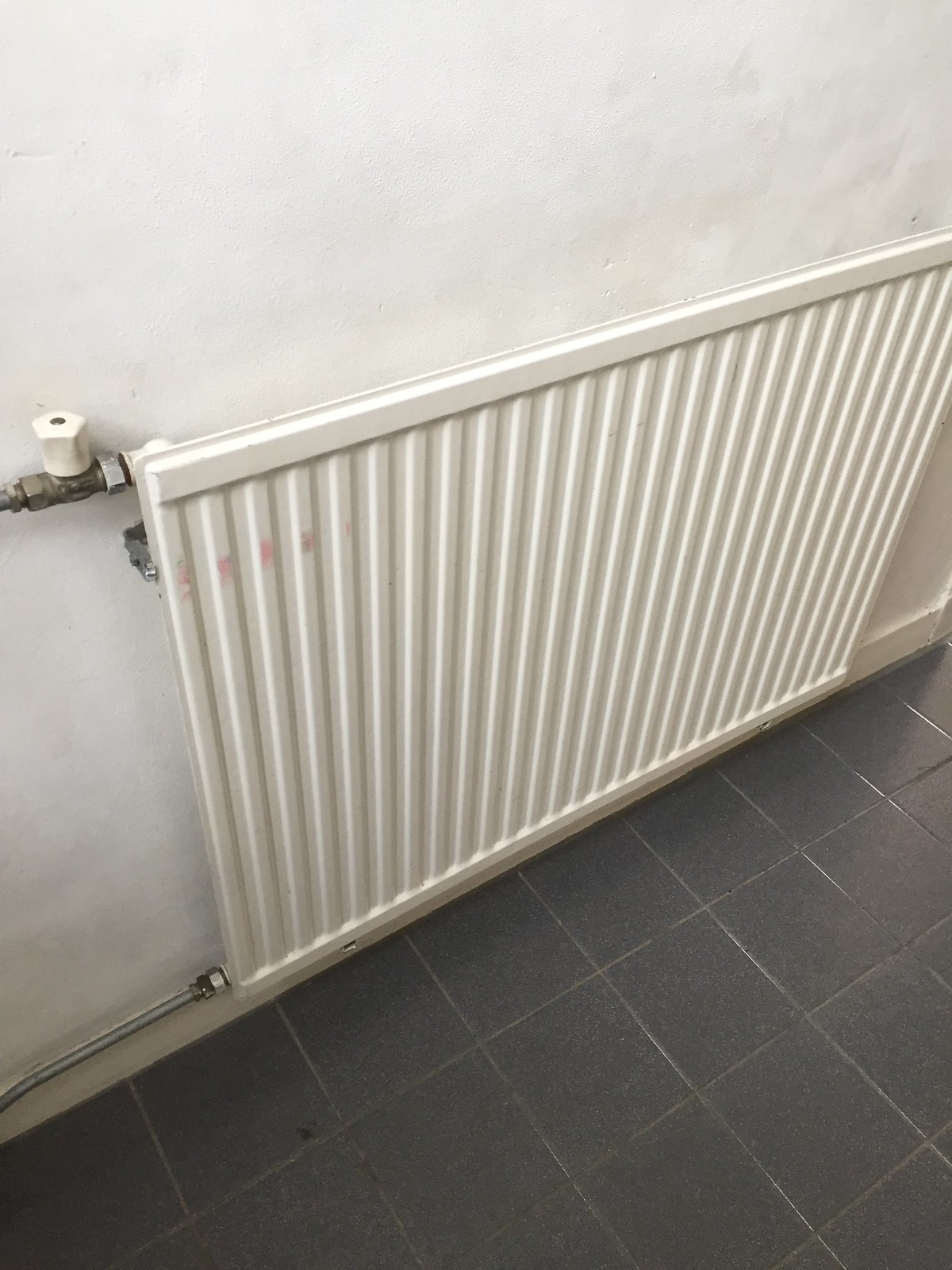The image captures a vertically rectangular view taken from an angle above, looking down the side of a white wall towards a tiled floor. The wall, which has noticeable dents and ridges, is adorned with a narrow, flat, white radiator that includes vertically grooved edges and a small pink streak. Extending from the radiator are pipes positioned at the top and bottom left, with one featuring a sizable, adjustable white screw—presumably for regulating the flow of liquid through the radiator. The floor below is covered with large, dark grey tiles, interspersed with hints of a deep brownish color and black, forming a pattern that leads diagonally from the lower left to the center right of the image. Additionally, the wall has molding at the bottom, adding a finishing touch to the uneven, patchy surface.